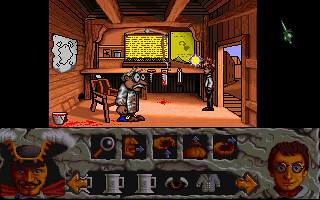A detailed still image from a retro video game captures a pivotal in-game moment. The top portion of the image showcases the gameplay scene, where the player character, a young child in a white shirt, has just entered a rustic wooden house. The child character stands before an archetypal scientist—an elderly man with white hair, clad in a classic lab coat. The scientist's wall is adorned with various texts and a prominent map, indicating important information or clues.

The lower half of the image features the game's user interface, likely an inventory or control panel. Key interactive options include a magnifying glass for examining objects, a speak option for dialogue, a hand icon for picking up items, and an open bag symbol for accessing inventory. Beneath these, there are various items available to the player. Additionally, the interface displays two decorative faces on the bottom left and bottom right corners, adding to the game's vintage aesthetic.